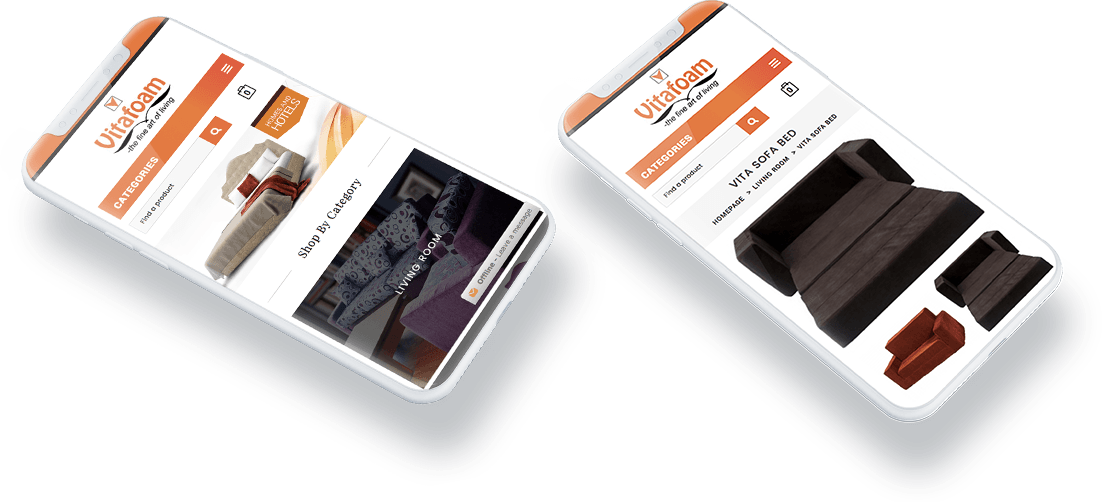The image showcases two illustrations of diagonal cell phone screens, each outlined without a border, set against a white background. The phone on the left leans slightly more to the left compared to the one on the right. Both screens cast a subtle gray or light gray speckled shadow toward their bottom-right edges.

Each screen displays the VitaFoam website. Below the centered VitaFoam logo, an orange gradient banner labeled "Categories" includes a three-bar dropdown menu. Directly beneath this banner is a "Find a Product" search box with an orange search icon button, accompanied by an indistinct icon.

On the left phone screen, two photographs are aligned vertically on the left side. The top photograph features a bed, next to which is an orange banner with text. This section is labeled "Shop by Category." Below it, a picture of a couch under a gray translucent screen bears the label "Living Room" in the center.

The right phone screen, beneath the same "Find a Product" search button, displays the text: "Vita Sofa Bed Homepage Living Room Vita Sofa Bed." This screen features three images of a fold-out sofa bed. The top image is a large, dark brown sofa bed. Beneath this, the left smaller image portrays a brick-red or dark orange couch in a non-folded state. The bottom right corner image replicates the large dark brown fold-out sofa bed but in a smaller size.